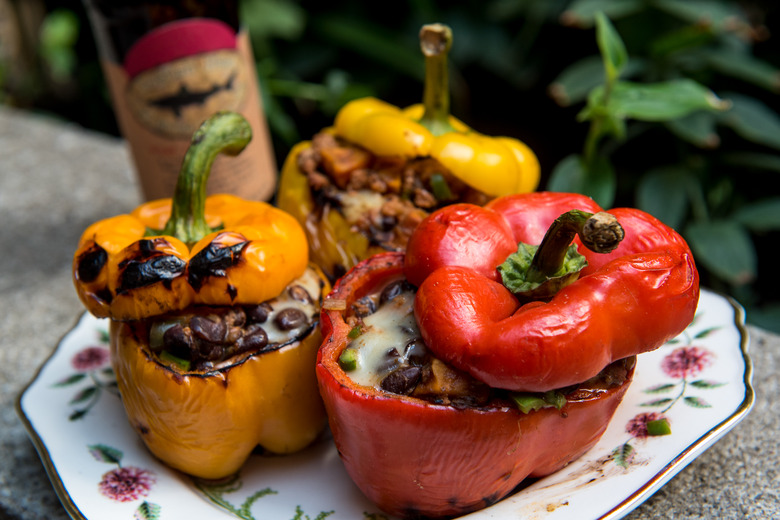This photograph showcases three stuffed bell peppers artfully arranged on an antique, white plate adorned with a pink and green floral pattern, further accentuated by an elegant gold rim. The dish includes a vibrant red pepper at the forefront on the right side, and two yellow peppers positioned towards the left and rear. The peppers, grilled to perfection as evidenced by the distinct caramelization marks, have their tops removed and are generously filled with a delectable mixture of cheese and beans, along with a possibly orange filling that could be pumpkin.

The setting, possibly outdoors, suggests a casual yet inviting atmosphere with green plants visible in the background. The plate is placed on what appears to be a stone or brick surface, enhancing the rustic charm of the scene. Accompanying these culinary delights is a bottle—perhaps of beer or wine—with a logo resembling that of Dogfish Head, adding a touch of sophistication. This elaborate presentation of grilled stuffed peppers suggests a hearty meal, likely meant for sharing, evoking the essence of summer dining.